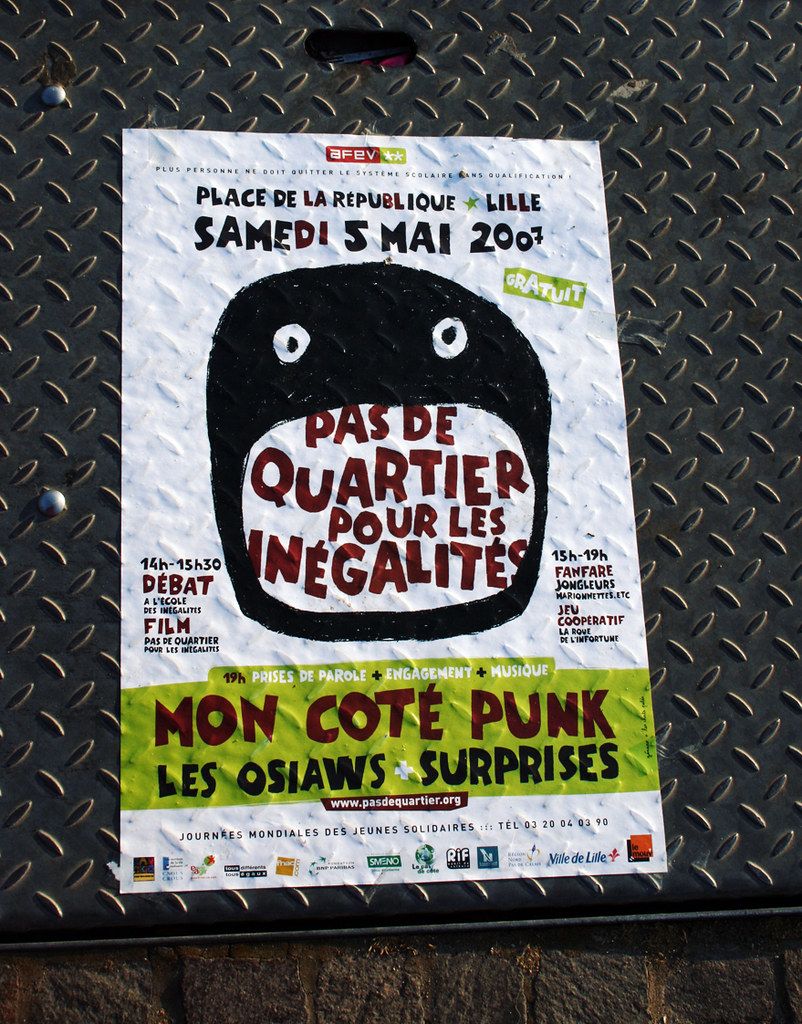The image features a promotional poster adhered to a black metal grate, which is mounted with flat head screws onto a rugged stone wall. The setting appears to be outdoors, given the natural lighting. The poster itself is primarily white, with a striking central illustration of a cartoonish black face with wide eyes and an exaggerated open mouth. Inside the mouth, in bold red text, the slogan "Pas de Quartier pour les Inégalités" is prominently displayed, translating to "No Quarter for Inequalities." At the top of the poster, "Place de la République Lille" is inscribed, followed by "Samedi 5 Mai 2007," indicating the event's location and date. Below the mouth, additional event information includes "Mon Cote Punk, Les Oswaldo plus Surprises," which likely refers to featured performances or attractions. The bottom section of the poster is filled with various logos, possibly representing sponsors or promoters. Notably, there is a green strip located at the bottom right-hand side of the poster, adding a small splash of color to the otherwise monochromatic design. The text and details suggest the advertisement is in French, targeting a French-speaking audience.